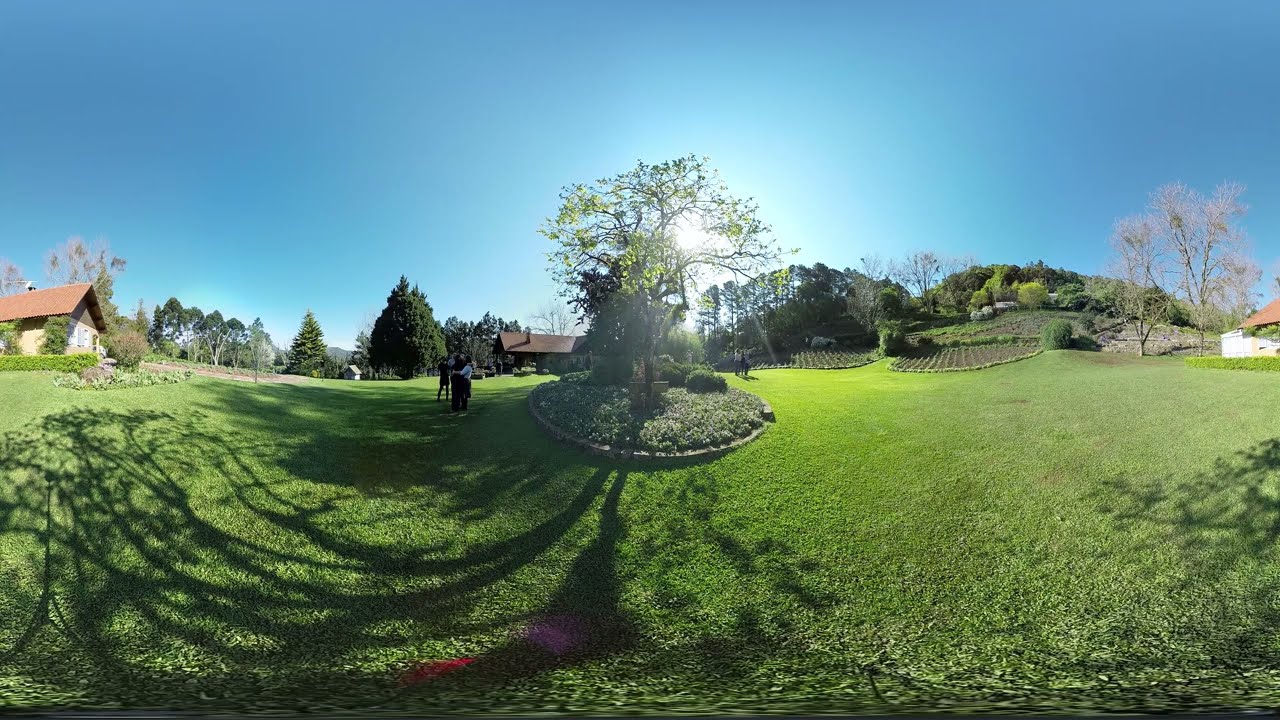The image depicts a vibrant, landscaped yard that appears to be captured with a fisheye or wide-angle lens, lending it a mildly distorted appearance. At the center is a circular garden bordered by bricks, containing a tall tree with sunlit green leaves and light purple flowers at its base. The sunlight filters through the leaves, casting distinct shadows on the cropped green grass. To the left of the tree, several people are visible, some seemingly embracing, and a house with an orange-tiled, sloped roof is situated further left. On the right, barren tall trees with only branches are seen alongside another partially visible house with a similar tile roof, backed by a hill with garden plots on it. The hill slopes upward towards a dense cluster of thick, leafy trees. The sky is a clear blue, becoming lighter near the sun. The overall scene is lush and green, creating a serene, picturesque setting that evokes the ambiance of a place suitable for meaningful gatherings or photo shoots.